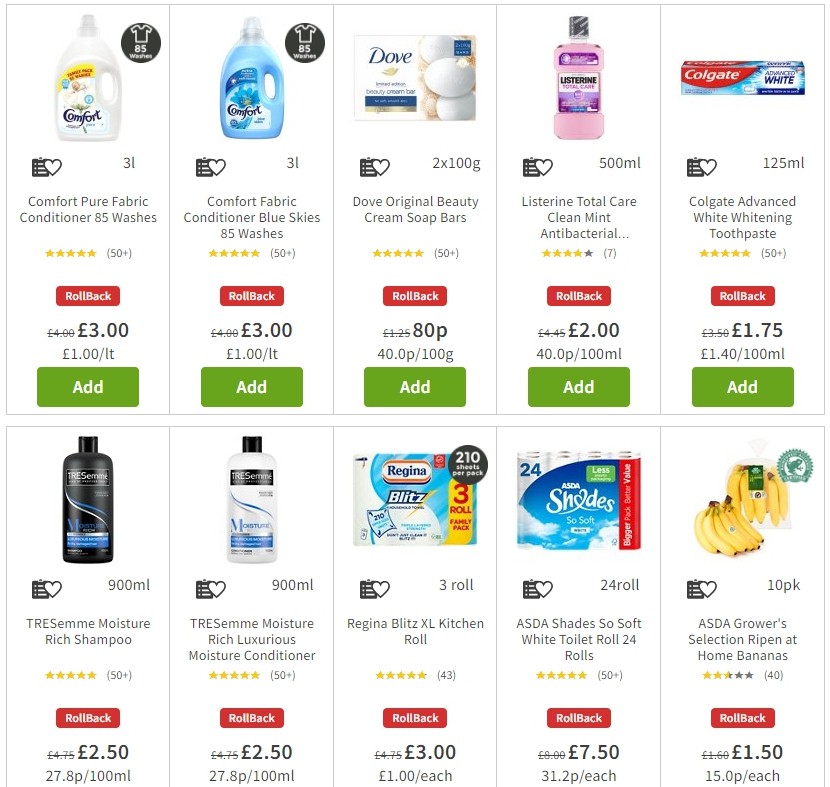This image is a detailed screenshot from an online store's last-second pop-up window, likely designed to prompt the shopper to add more items to their order before checkout. The screenshot showcases a selection of various products, each accompanied by a green "Add" button. Among the items displayed, there is a range of personal care and household products, including toothpaste from Colgate, mouthwash from Listerine, a bar of soap from Dove, a bottle of Tresemme shampoo, and Tresemme conditioner. Household essentials like laundry detergent, a bunch of bananas, and packs of toilet paper are also visible. Each product is individually priced in pounds, with prices varying from as low as £0.80 to as high as £7.50. The clear, detailed layout allows the shopper to see all the available items and their prices at a glance, encouraging additional purchases just before completing the transaction.